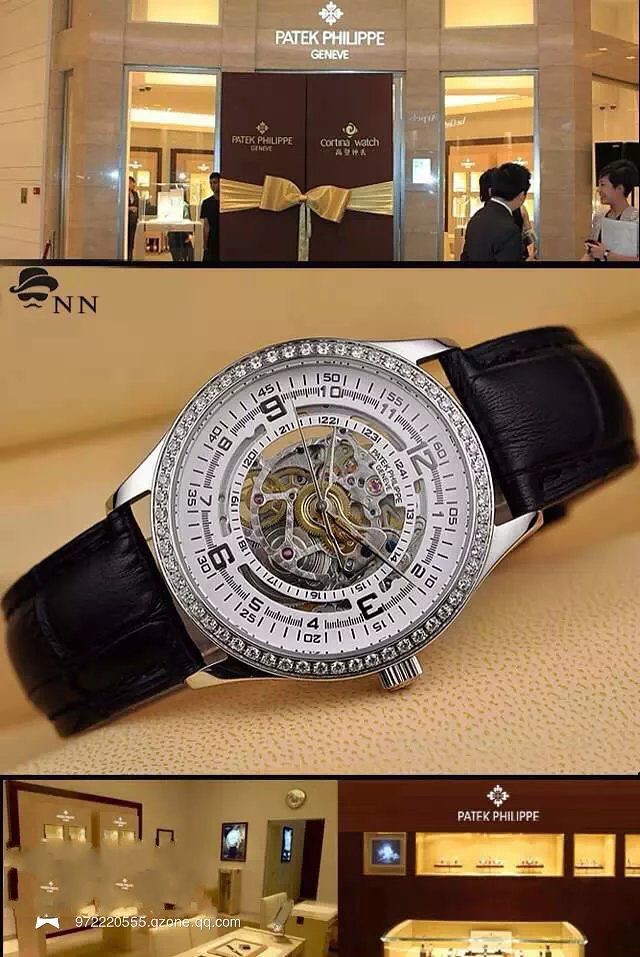The image is a vertical collage of three distinct photographs depicting various aspects of a high-end watch store. The top section, occupying about a quarter of the page, showcases the exterior of a luxurious store named "Patek Philippe" located in Geneva. The storefront has a brown facade with a large window that offers a glimpse inside. There's a brick-like border adorning one side, and visible above the window is a smaller pane. Prominent red double doors, tied with a yellow ribbon bearing indistinct white lettering, suggest that it might be a grand opening. The name "Patek Philippe" is emblazoned above in large lettering, with "Geneve" noted beneath it. In front of the window, a man with black hair, dressed in a suit, stands in conversation with a woman who has short black hair, a white shirt, and holds a piece of paper.

The middle portion, which takes up about half the page, focuses on an intricate, expensive-looking watch. The watch features a black leather strap and a face that is silver and white, bordered by a ring of small diamonds. The design is modern and showcases the inner workings of its mechanical elements through the transparent face, revealing a detailed assembly of gears and numbers.

The bottom quarter of the page is divided into two images. The left side displays an interior view of the store, highlighting various jewelry displays and cases, likely showcasing items such as earrings and other timepieces. The right section features a red display case marked with the Patek Philippe insignia at the top and plaques on the surrounding walls. An additional watermark reading "gzone.qq.com" and a long number is faintly visible in the image's corner.